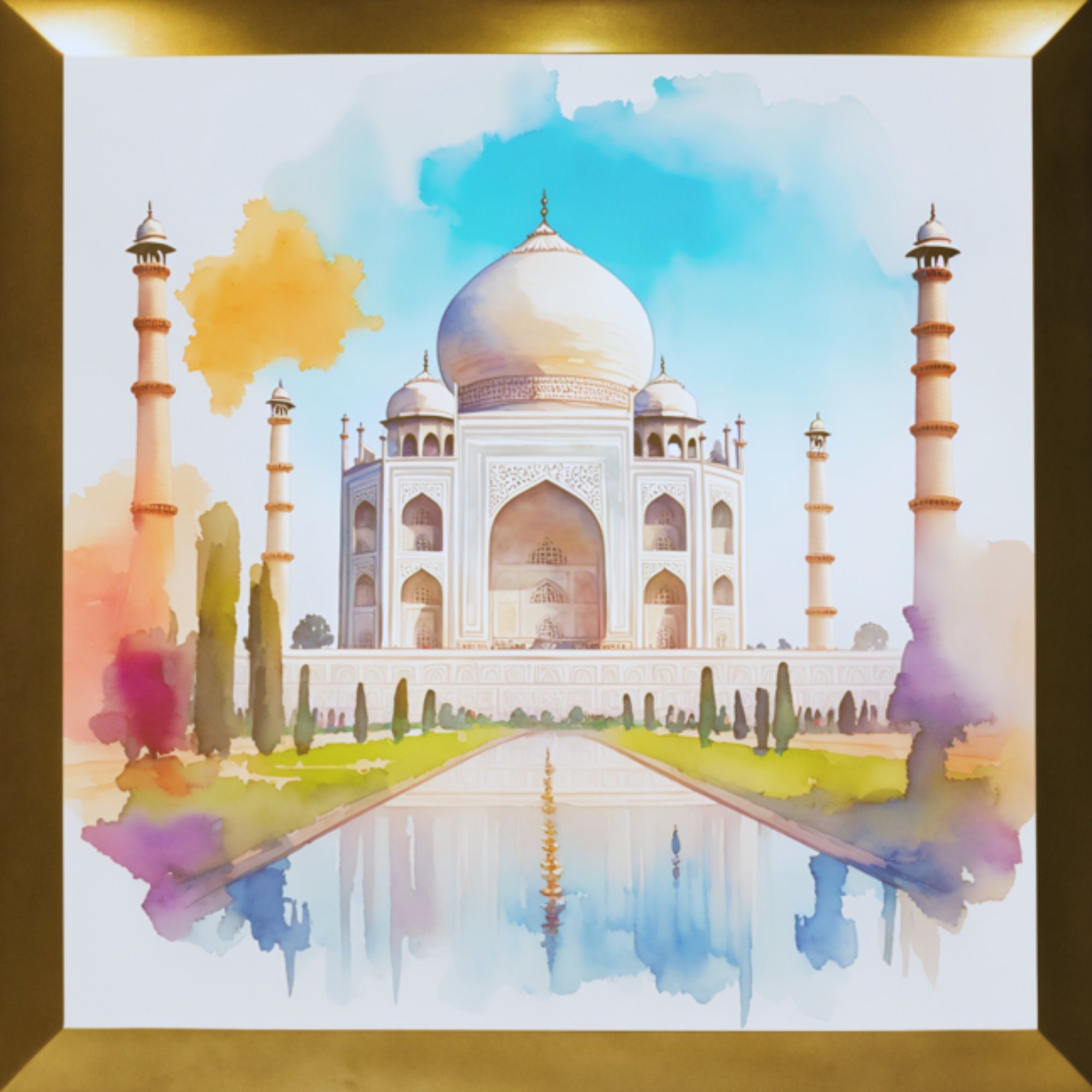This detailed watercolor painting captures the iconic Taj Mahal with an artistic flair that blends realism with abstract elements. The central focus is on the Taj Mahal itself, rendered in various beige tones, its grand central dome flanked by two smaller domes and surrounded by four cylindrical towers, each topped with a smaller dome. The palace is reflected in a mirror-like water pool in the foreground, with green lawns and splotchy trees on either side, adding depth to the scene. The sky, painted in shades of blue with yellow-tinged clouds and occasional blue and purple accents, enhances the overall vibrant composition. An ornate, gold-colored frame, likely added digitally, surrounds the artwork, contributing to its elaborate and fancy appearance reminiscent of a gilded palace like the one in Aladdin. The image overall combines detailed architectural depiction with abstract, free-flowing watercolor techniques, creating a visually striking and colorful representation of this iconic monument.